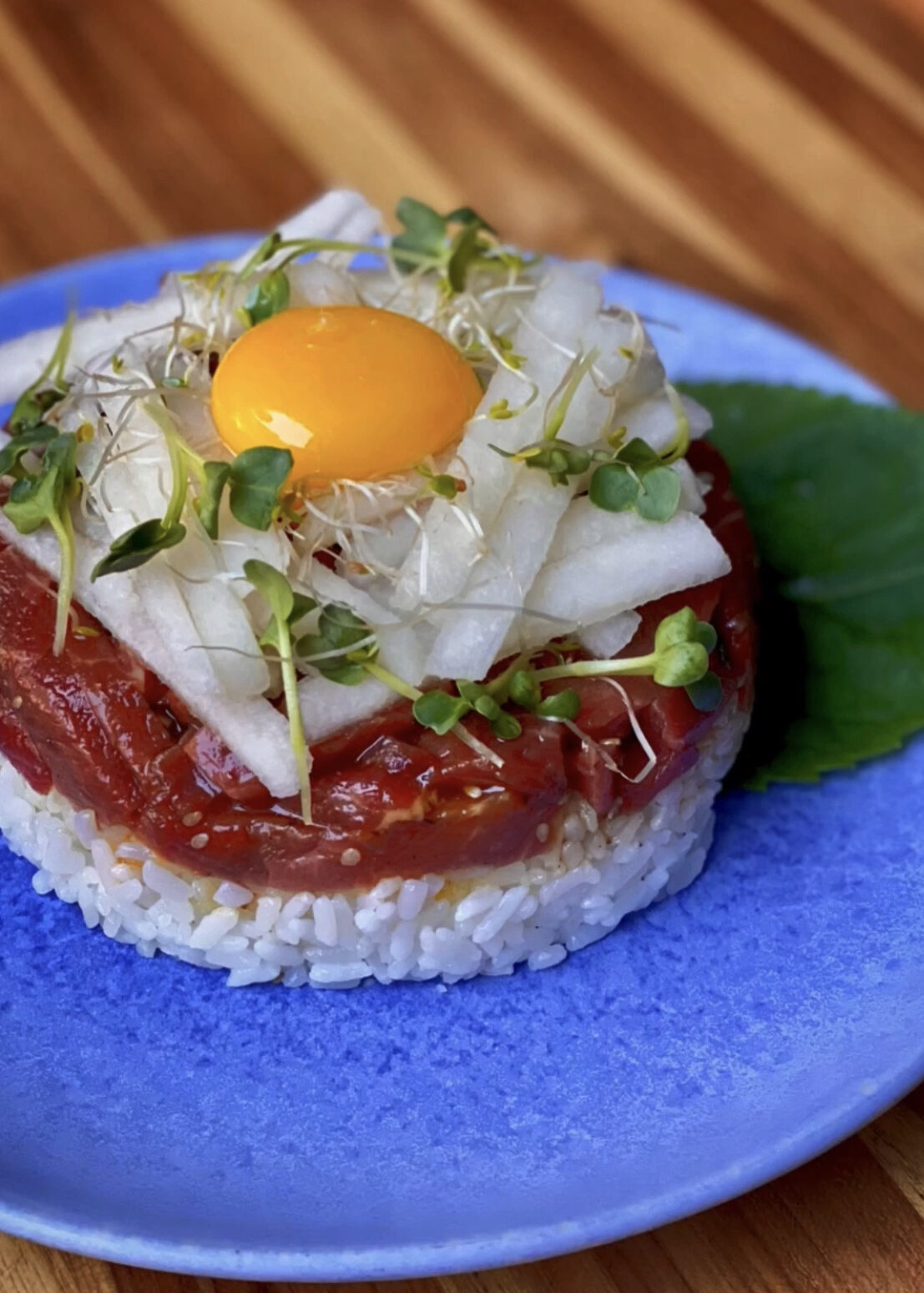The image showcases a beautifully arranged Japanese-inspired dish served on a periwinkle-speckled blue plate. At its base is a meticulously shaped patty of white rice. Topping the rice is a layer of raw red fish, fashioned into a similarly shaped patty. This is adorned with thin, crisp white strips that could be either onions or white daikon radish. Further accentuating the presentation, microgreens, and possibly root greens, are scattered atop the dish, providing a burst of fresh color. Crowned majestically at the peak of this culinary creation is a glossy, golden raw egg yolk. A single green round leaf garnish is positioned on the top left of the plate, adding an extra touch of artistry. The plate itself is placed on a light wooden table with visible vertical lines from the wood planks, enhancing the natural and inviting feel of the overall presentation.